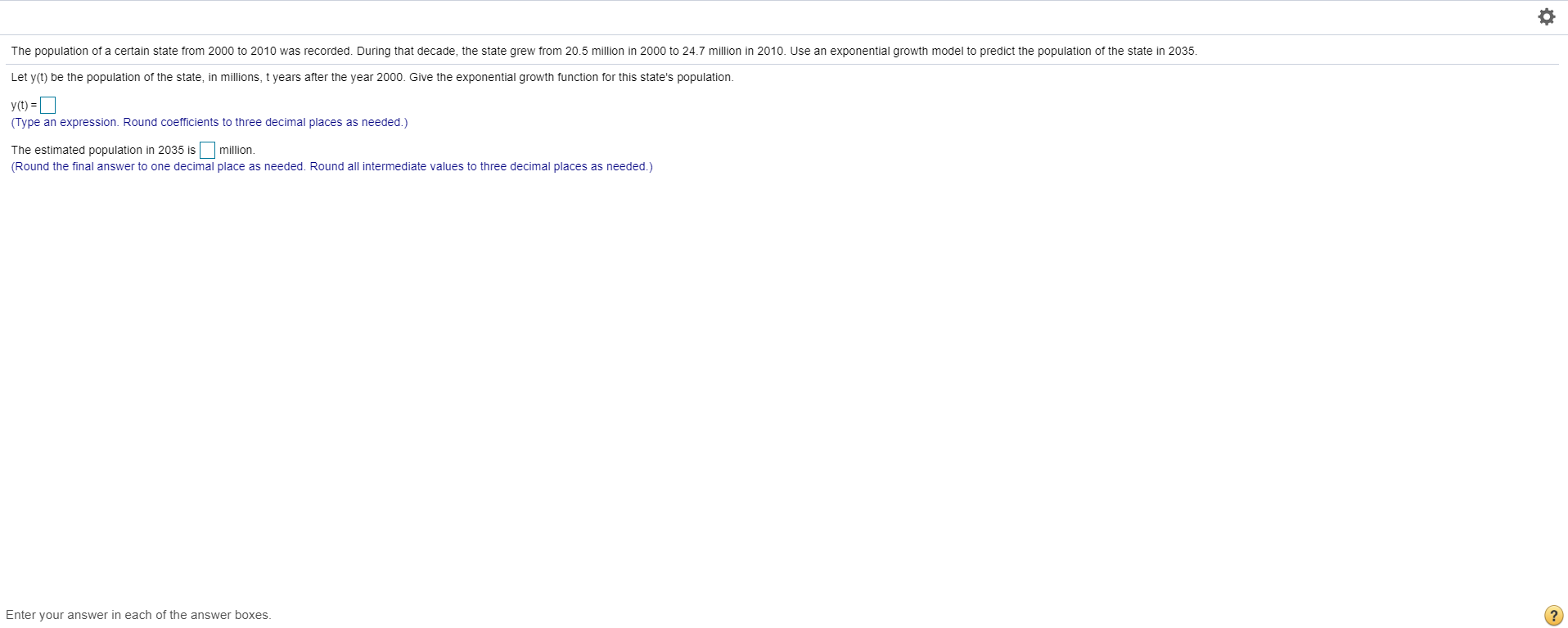The image is a screenshot of a webpage displaying a population growth task for a state between the years 2000 and 2010. In very small print at the top, it notes that the state's population grew from 20.5 million in 2000 to 24.7 million in 2010. The task includes using an exponential growth model to predict the population of the state in 2035. 

The instructions mention defining \( Y_t \) as the population of the state, in millions, \( t \) years after the year 2000. The task requires formulating the exponential growth function to describe this population change, denoted as \( Y_t = \) [expression to be typed], with coefficients rounded to three decimal places as needed. 

Furthermore, it specifies that the estimated population in 2035 should be entered into an empty square provided, with the result in millions. The final answer should be rounded to one decimal place, and all intermediate values should also be rounded to three decimal places as needed. 

The central part of the image is predominantly white space, with a small message at the bottom instructing users to enter their answers in the boxes provided. There is a yellow circle with a blue question mark on the right side for any questions or additional help.